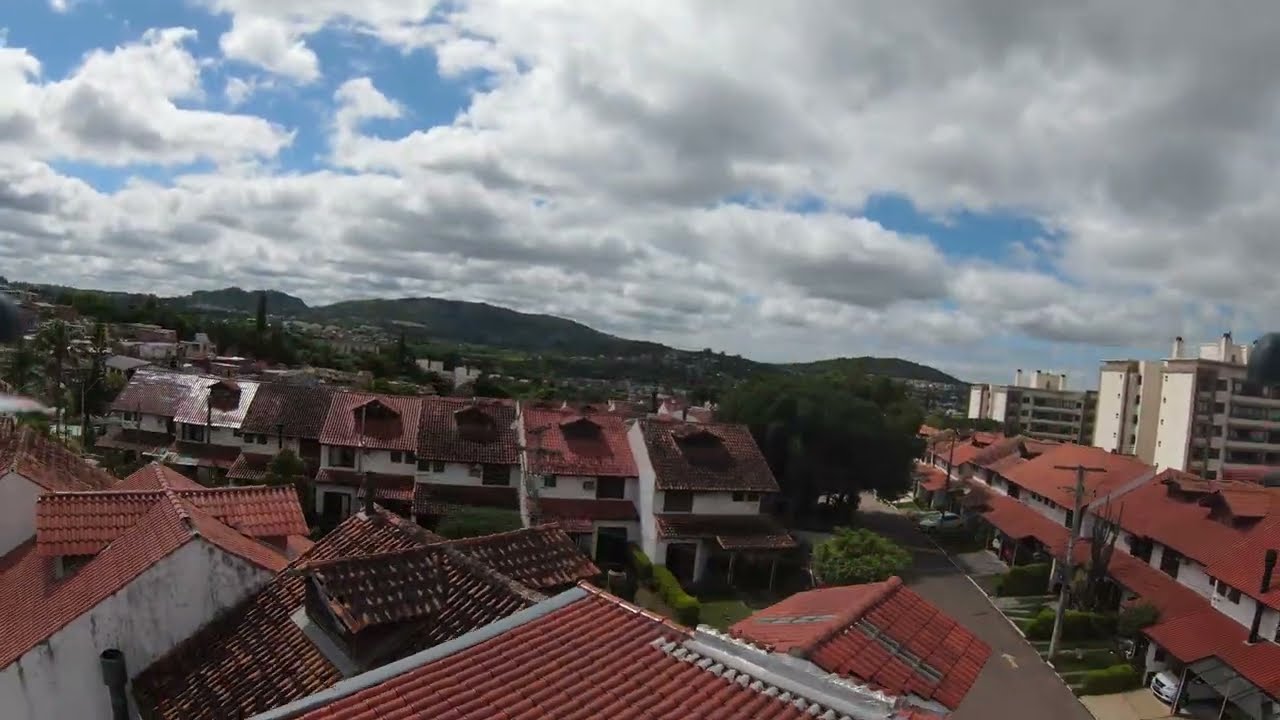The photograph showcases a suburban cityscape, potentially somewhere in Europe, captured from a rooftop perspective. The top half of the image is dominated by a blue sky interspersed with an abundance of fluffy white clouds, suggesting a partly cloudy day. Below this expansive sky, the horizon reveals distant mountains or elevated terrain that appears brownish, adding a natural backdrop to the urban foreground. 

In the middle and foreground sections, the city is a mosaic of residential buildings, predominantly white townhouses and condos with red tile or shingled roofs, arranged in a somewhat triangular formation. These dwellings reflect an old-style architectural charm. Visible details include green trees scattered among the buildings, adding a touch of nature to the urban setting. 

To the right side of the image, the scene transitions downwards, revealing a street lined with more homes and some taller white buildings that resemble condominiums or hotels, with multiple levels visible. A few cars are also discernible on the streets. The photograph effectively captures the essence of this quaint, suburban landscape, framed by the distant mountains and under a sky dotted with clouds.